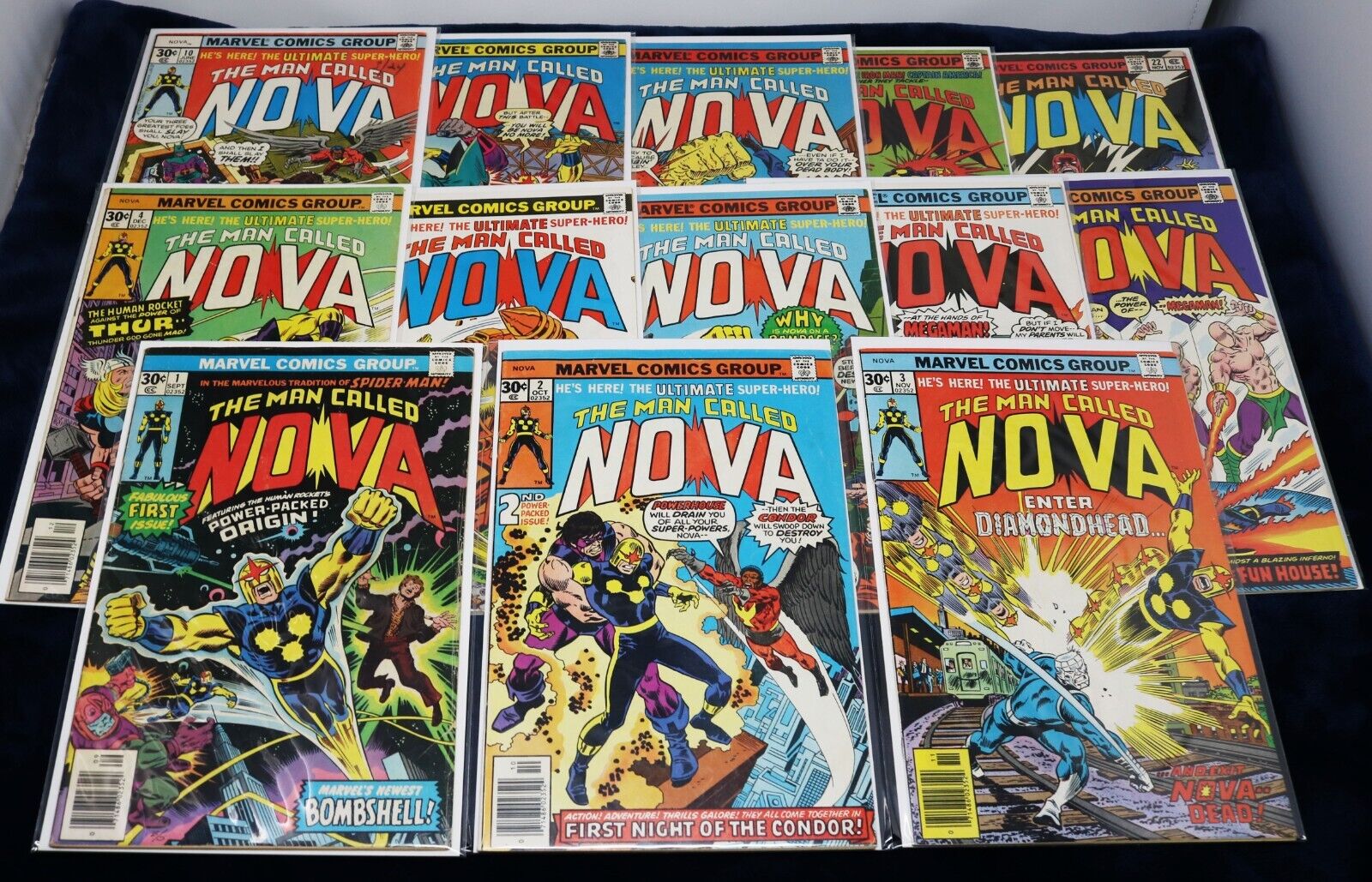A collection of thirteen vintage comic books is meticulously displayed on a small table. The comics are organized in three neat rows: five on the top row, five in the middle, and three on the bottom. Each comic cover prominently features the title "Nova" in various striking color combinations such as white and blue, red and white, white and red, and red and black. The top of each cover reads "Marvel Comic Group," and beneath that, the phrase "He's here, the ultimate superhero. The man called Nova" announces the hero's presence. The covers are vibrant and visually captivating, showcasing a palette dominated by yellow, blue, and red hues.